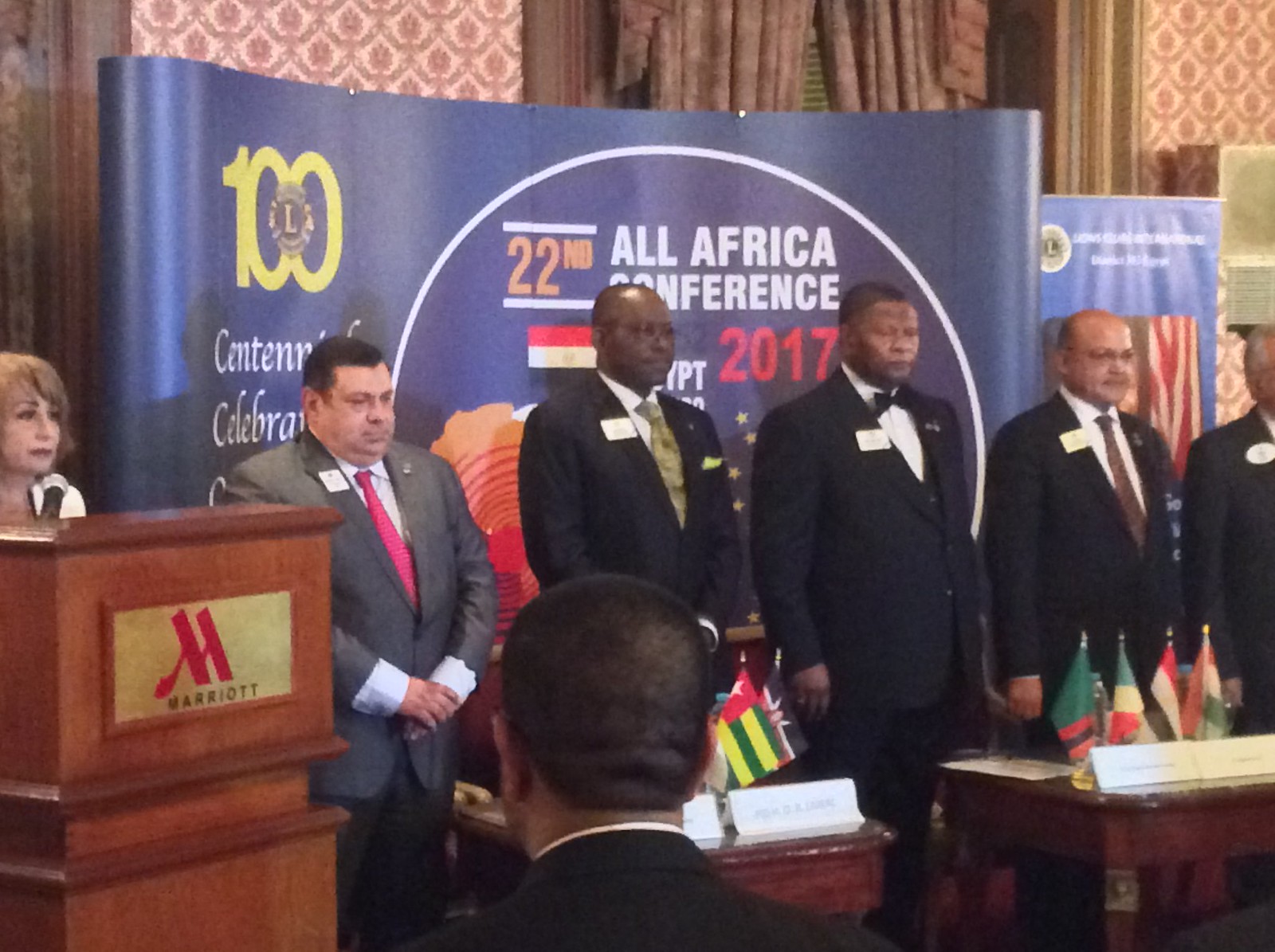This photograph captures a formal scene from the 22nd All-Africa Conference held in 2017 at the Marriott Hotel. At the forefront, seven individuals are lined up, positioned in front of a banner displaying the conference name. A woman stands behind a podium emblazoned with the Marriott logo, holding a microphone, while the six men beside her are dressed in suits and ties, with one donning a bow tie. Each participant wears a sticky name tag affixed to their suit. In front of this assembly, tables are neatly arranged with small flags representing various countries and corresponding name tags. These are small, standing tables rather than round sit-down ones. The room itself is elegantly decorated with wallpaper and large drapes, creating a sophisticated backdrop for this diverse group of attendees.